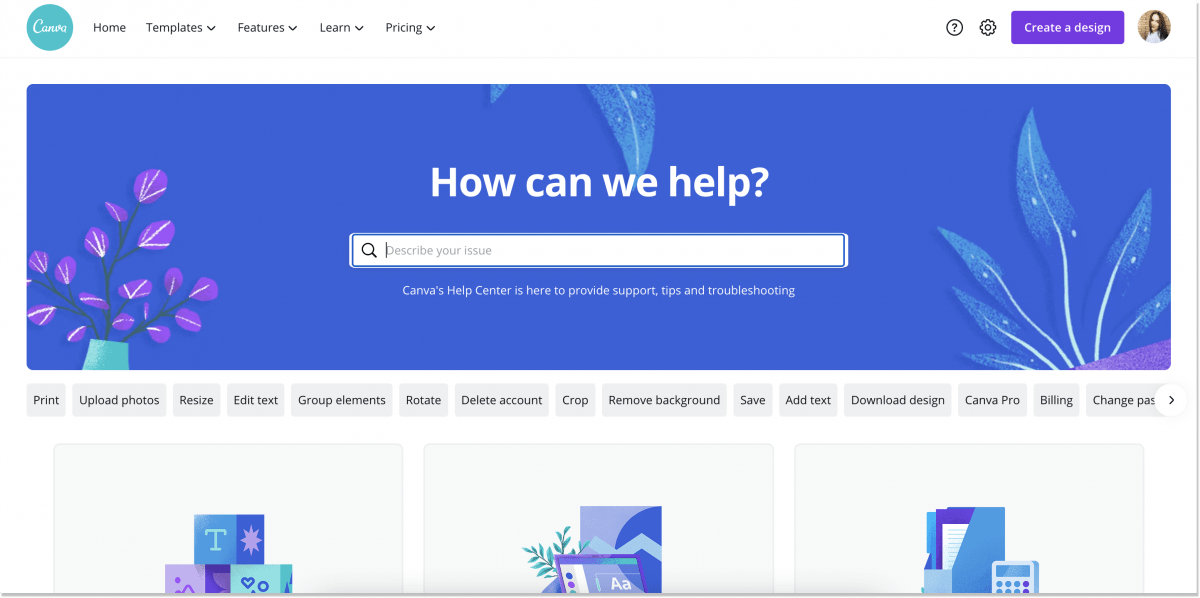The image appears to be a screenshot of a Canva webpage. At the very top, there is a white border. In the left corner, a small blue circle contains text that is too tiny to read, but it likely says "Canva." To the right of this circle, the navigation bar displays the following options: Home, Templates, Features, Learn, and Pricing. On the far right of the navigation bar, there is a question mark icon inside a circle, a gear icon, and a purple "Create a Design" button adjacent to a circular profile picture of a female.

Beneath this top border, the background transitions into a blue color with a large purple flower on the left and some green wavy leaves adjacent to it. Centered on the right side, bold text reads "How can we help?" directly above a search bar. Below the search bar, additional text states, "Canva's Help Center is here to provide support, tips, and troubleshooting."

Further down, under this section, there are additional options listed: Print, Upload Photos, Resize, Edit Text, Group Elements, Rotate, Delete Account, Crop, Remove Background, Save, Add Text, Download Design, Canva Pro, Billing, and another option that is partially cut off. 

At the bottom of the image, there are three incomplete square icons. The first appears to feature blocks or a grid, the second possibly represents a computer, and the third icon shows what appears to be a file and a calculator.